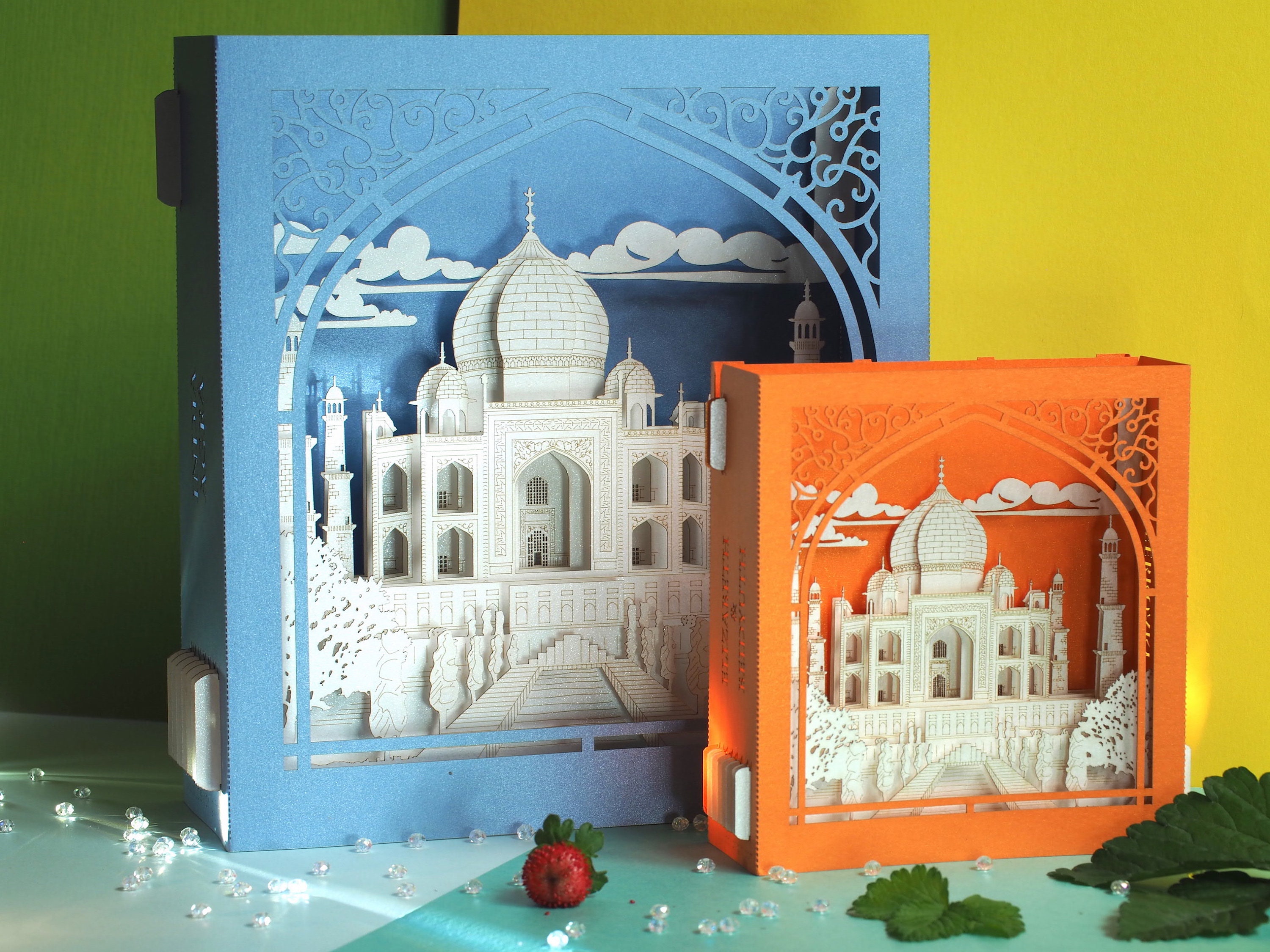In the image, we see two intricately crafted papier-mâché models of the Taj Mahal, both adorned with detailed etchings of elements such as white clouds, trees, and steps leading up to the iconic structure with its central dome flanked by four towers. The larger model is housed within a blue-framed box, while the smaller, identical version resides in an orange-framed box. These models are placed against a backdrop featuring green and goldish-yellow walls. They sit on a multi-toned blue table, which is scattered with small, clear crystals and green leaves. A lone strawberry, positioned centrally, adds an unexpected whimsical touch to the scene. The combination of these elements creates a visually striking and meticulously detailed arrangement, emphasizing the grandeur and symmetry of the renowned architectural marvel.